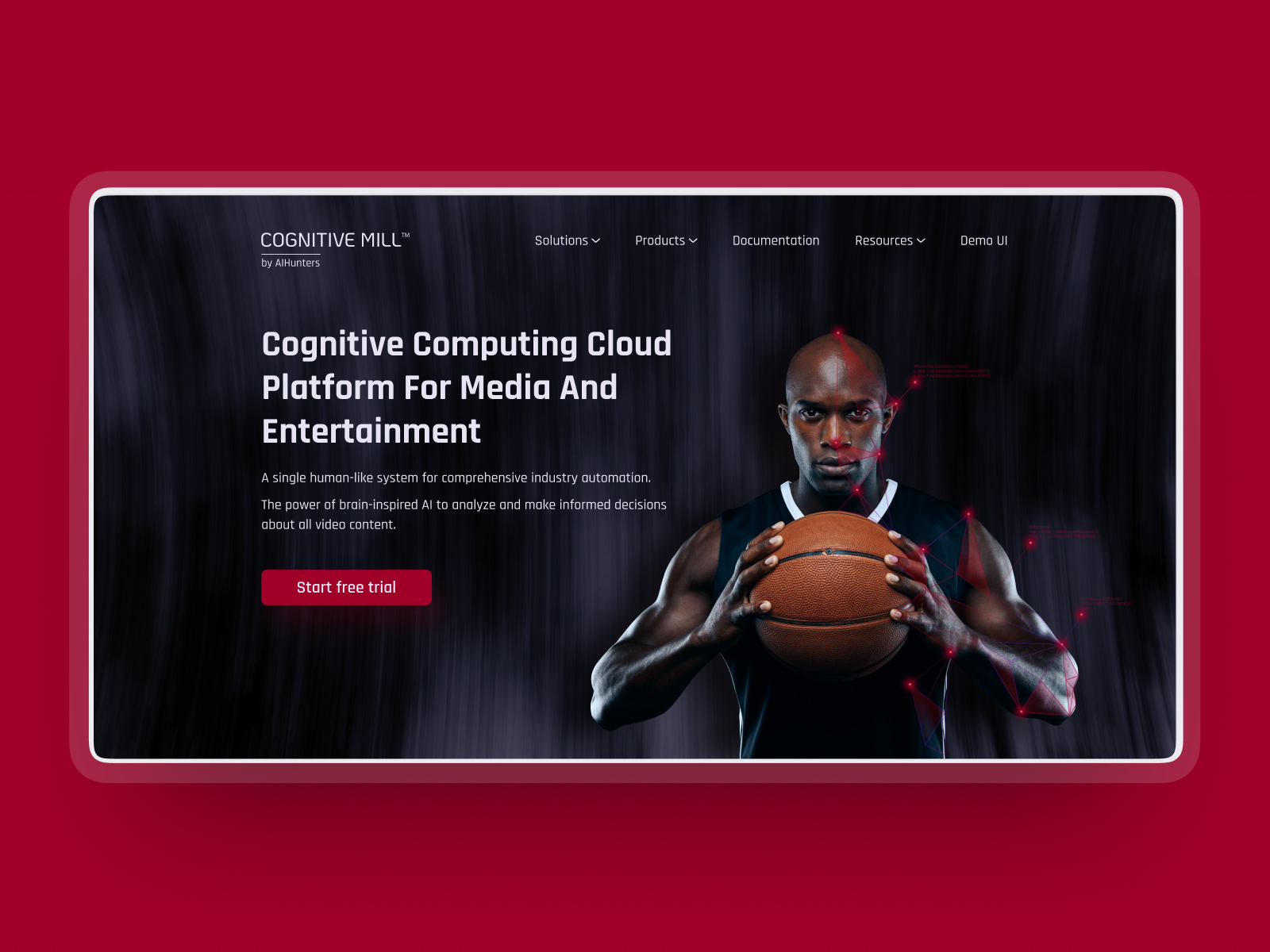In this rectangular image set against a vibrant red background, we see a high-resolution, color screenshot of a young African-American male basketball player on the right side. The athlete, depicted waist-up, has a muscular build and a shaved head. He faces forward with an intense, serious expression, and his mouth is closed. His elbows are out as he firmly grips an orange and black striped basketball with both hands. Small red dots of light are visible along the right side of his body, adding to the intense ambiance of the image.

To the left of the player, bold white text over a black and gray backdrop reads, "Cognitive Computing Cloud Platform for Media and Entertainment." Below this text, there is a prominent red button inviting viewers to "Start Free Trial."